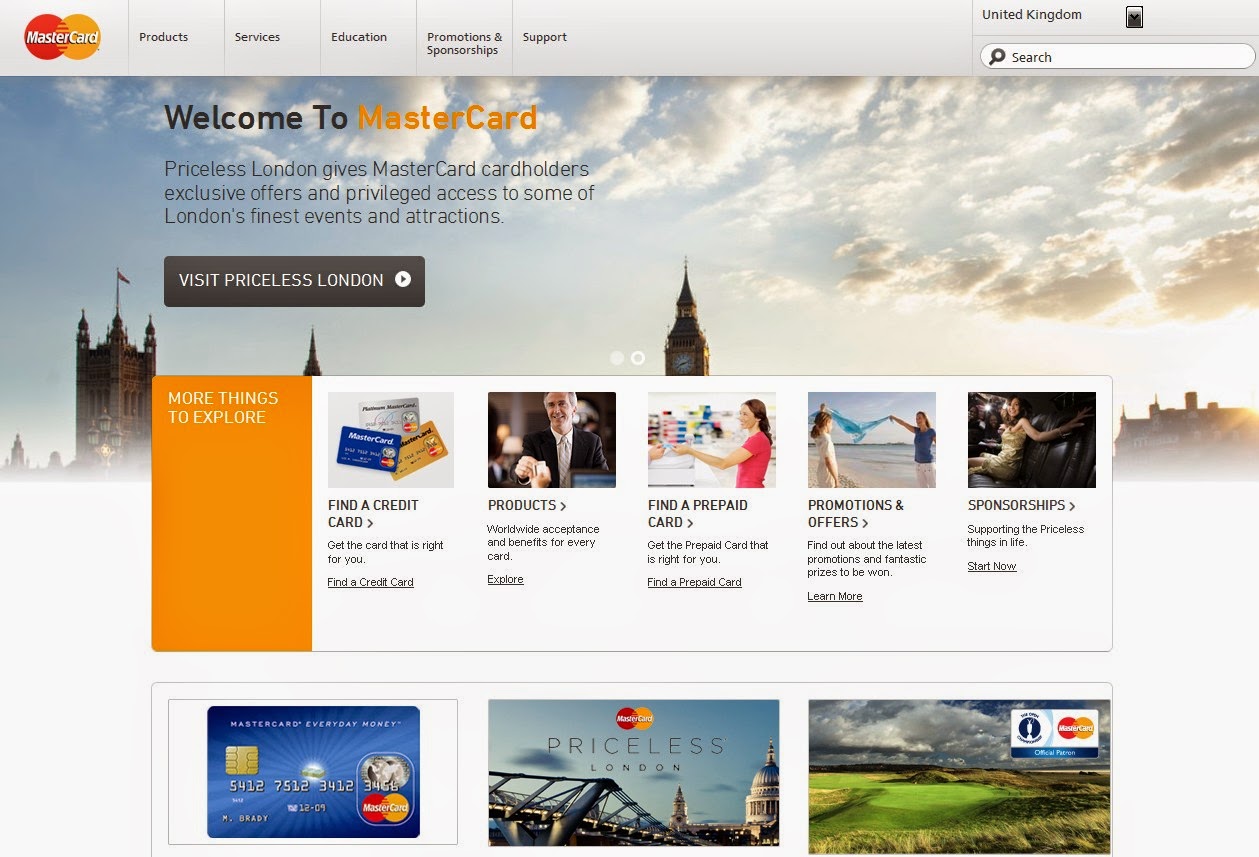Screenshot of the MasterCard UK Website

The image captures a prominent screenshot from the MasterCard website tailored for the United Kingdom. The top of the page features the iconic MasterCard logo, immediately identifiable with its overlapping red and yellow circles. The primary navigation menu offers a variety of options: Products, Services, Education, Promotions, and Sponsorship, each designed to guide the user through MasterCard's offerings.

A key detail on this page is the location indicator at the top, specifying that the site’s content is localized for the United Kingdom. One notable button, labeled "Priceless London," suggests exclusive features and experiences available specifically within London. In the background, a captivating image of the London skyline sets a compelling scene, showcasing landmarks like the Elizabeth Tower (commonly mistaken as Big Ben, which is actually the bell inside the tower) and another recognizable structure, possibly The Shard. The sky is overcast with clouds, hinting at a typical London weather scene, while the sun sets off to the right, casting a warm glow over the city.

Further down, the submenu offers additional options for deeper exploration: users can find various credit card products, locate a prepaid card, look into current promotions, and review sponsorship opportunities. Decorative images at the bottom of the page display different card designs, including a special edition card themed "Priceless London," adorned with a picturesque view of the London skyline.

This descriptive caption provides a detailed yet concise overview of the webpage, emphasizing the localized content and visually appealing elements specific to London's culture and iconic imagery.